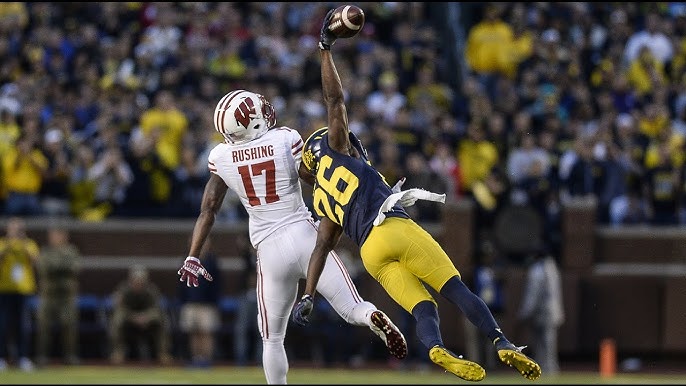This is a color photograph capturing an intense moment in a football game, oriented horizontally with a blurred stadium background full of spectators. The image features two African American players in action. The player on the left is wearing a white helmet with a red "W" on the side, a white jersey with the name "RUSHING" and the number 17 in red lettering, white pants with red stripes, and red gloves. His leg is kicked up behind him as he presumably tries to defend against or catch the football. The player on the right, who appears to have the ball in his left hand, is dressed in a dark blue uniform with yellow accents, a dark blue helmet with yellow detailing, a dark blue jersey with the yellow number 26, matching dark blue socks, yellow pants, and yellow cleats. He also has a towel hanging from his waistband. The scene suggests a pivotal play, possibly involving a catch or a defensive maneuver, creating a dynamic and engaging moment captured on the field.